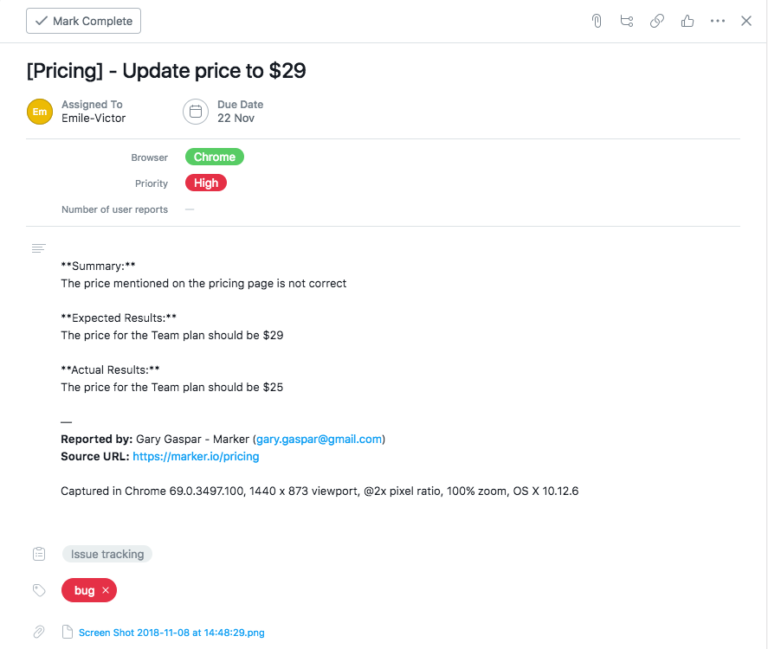The image displays a structured task summary:

1. In the top left corner, a checkmark is accompanied by the text "Mark Complete" and both are underlined with a long, light-gray line.
2. Below this, in parentheses, is the word "Pricing," followed by a small dash and the update directive "Update price to $29."
3. This task is assigned to "Emil-Victor" with a due date of "22 November."
4. Next, a long line separates the above section from the following details.
5. The word "Browser" appears, with "Chrome" enclosed in a green circle beside it.
6. Below "Browser" is the term "Priority." To its right, in a red circle, the word "High" (H-I-G-H) is displayed.
7. Further down, "Number of User Reports" is mentioned.
8. Another separating line follows, leading to the sections "Summary," "Expected Results," and "Actual Results."
9. In black text, the task is reported by "Gary Gasper" with the marker information. His email "gary.gasper@gmail.com" is listed in blue.
10. The "Source URL" is provided in blue text: "https://marker.io/pricing."
11. At the bottom, a red circle encloses the word "Bug," followed by an 'X.'
12. Finally, at the very bottom, the date "Screenshot 2018-11-08" is displayed in blue text.